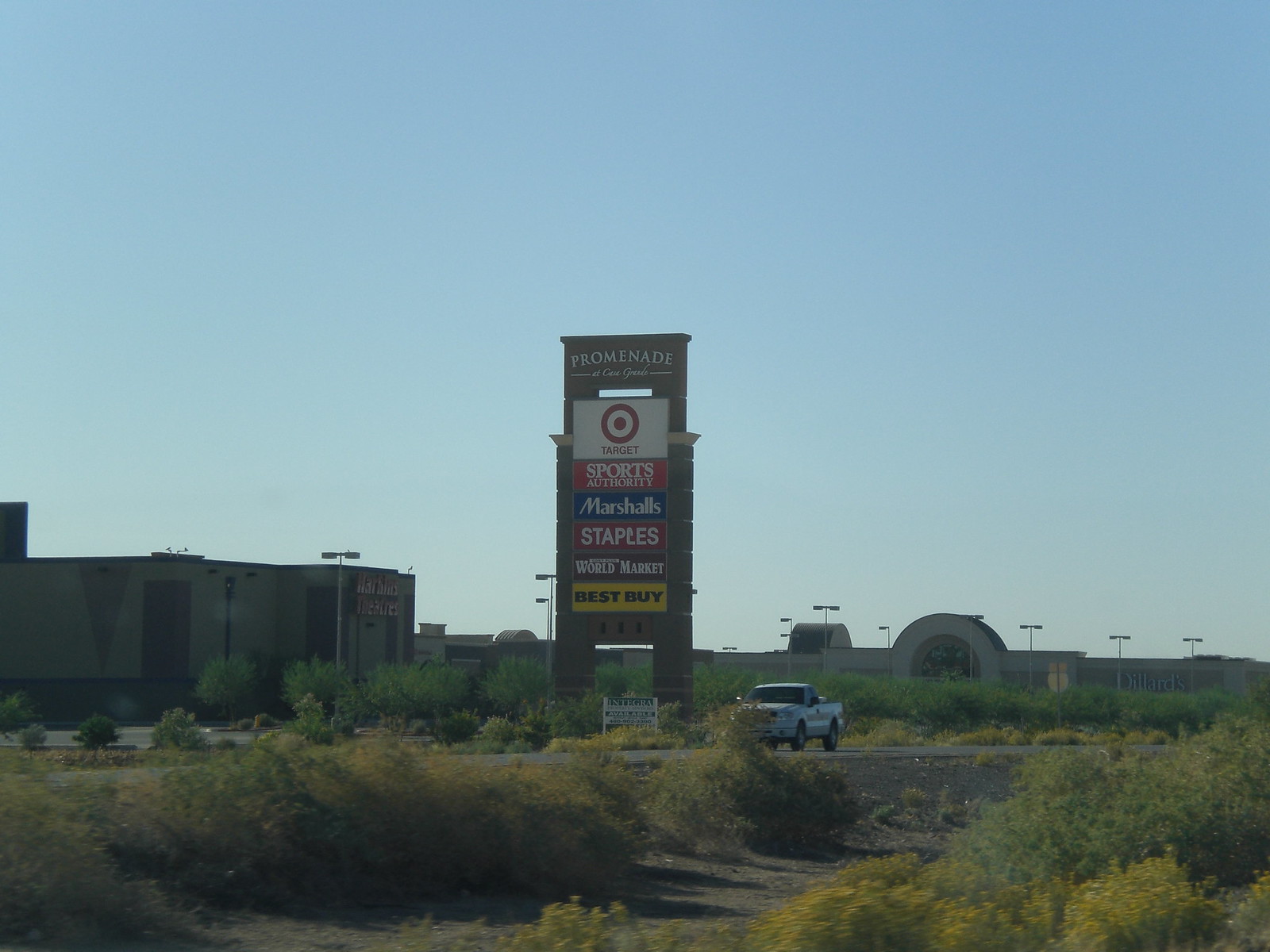A panoramic view of Promenade Industrial Estate, a commercial park, stretches across a landscape of scrubland. Dominating the scene is a towering sign that names the estate and showcases several prominent retailers, including Sports Direct, Marshalls, Staples, and Best Buy among others. Running through the center of the image is a busy highway, featuring a white half-truck in motion. To the left, stands a collection of square, utilitarian buildings, while an archway marks the entrance to the shopping complex. The gateway frames additional structures visible in the background. The blue sky overhead provides a vibrant contrast to the green shrubbery scattered throughout the foreground, painting a lively backdrop for this bustling commercial hub.